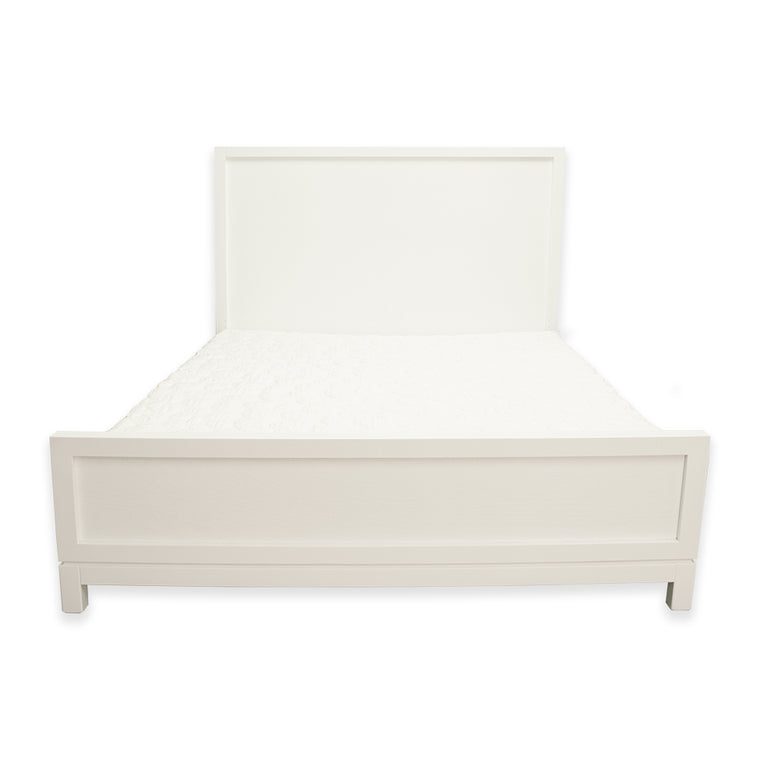This image depicts a simple, minimalist white bed frame set against a completely white background. Notably devoid of any mattress or bedding, the frame itself becomes the primary focus. The bed frame is constructed from off-white wood, characterized by clean lines and a broad rectangular base that contains a smaller carved-out rectangle. This structure is supported by thick wooden legs, capped with tiny posts at each end. The flat surface of the bed frame narrows in perspective as it rises, converging towards the top. Dominating the upper portion of the image is a tall, rectangular headboard made from the same off-white wood, bordered in a similar style to the base. This detailed design element contributes to an overall sense of symmetry and solidity, offering a sturdy yet elegant piece that appears well-suited for a queen-sized mattress, though none is present.